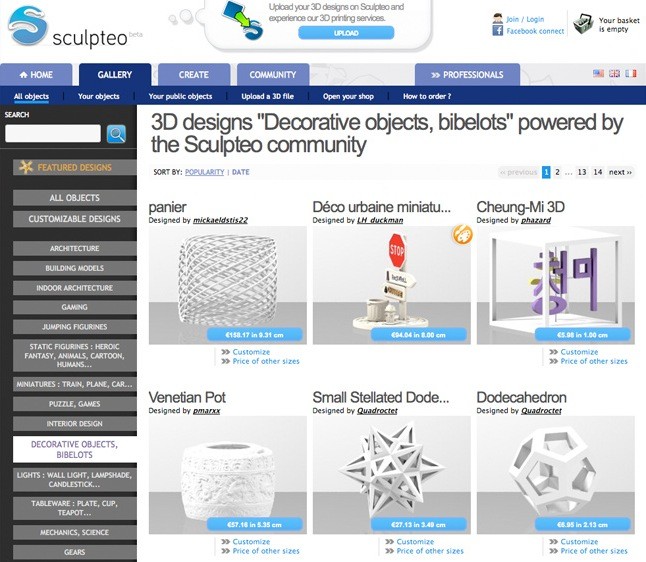This screenshot from the Sculptio Better website features a prominently displayed logo in blue and white, depicting a highly stylized, 3D-rendered letter "S." A speech bubble emanating from the logo invites users to "Upload your 3D designs on Sculptio and experience our 3D printing service." In the top right corner, there are options for "Join," "Login," and "Facebook Connect," indicating different ways to access the website's services. The shopping basket icon shows it is currently empty, suggesting no items have been purchased yet.

On the left side of the page, a variety of products are listed, including a 3D printed pannier and a Deco Urban miniature, the latter described in French. The website showcases designs created by various members of the Sculptio community, who likely offer their creations for sale. Categories on display include games, puzzles, lights, gears, and jumping figurines, illustrating the diverse range of 3D-printed items available.